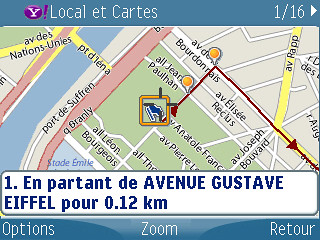The image is a detailed section of a Yahoo Maps interface, presented in French, focusing on the general area around the Eiffel Tower. The top of the map features blue-bordered edges containing Yahoo's logo—a purple circle with a white "Y" and an exclamation mark, followed by the text "local et Cartes" in white. On the right side of this bar, it reads "1 of 16" with a right-pointing arrow to change map views. The bottom blue border includes white text reading "Options, Zoom, and Retour," indicating additional functionalities. 

The map itself is vividly colored, showing various geographic elements such as waterways to the left, marked with blue, and a network of roads—yellow bridges, red road outlines, and green spaces. Significant streets and points of interest are highlighted in orange and other shades, with street names prominently displayed. A specific point of reference at the bottom indicates "No. 1" and mentions the Eiffel Tower in French ("Tour Eiffel"), accompanied by "En partant de Avenue Gustave" among other details.